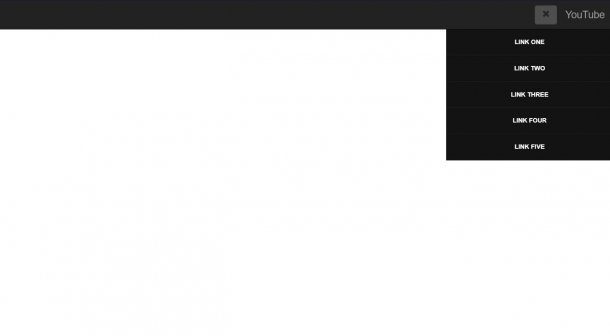The image showcases a website interface featuring a prominent horizontal black navigation bar spanning the top third of the page. Below this bar, the background is stark white and devoid of any text or imagery. In the black bar, there is a recognizable text field where users can presumably enter a URL, though there is no visible cursor. On the right-hand side of this bar, there is a rectangular box with an 'X', suggesting a cancel or close function. Adjacent to this box, the word "YouTube" is displayed in its distinctive font and layout. Directly beneath the main black bar, there's a drop-down menu listing five selectable links: 'Link 1', 'Link 2', 'Link 3', 'Link 4', and 'Link 5'. Each link appears clickable, likely directing users to different sections or pages associated with YouTube.